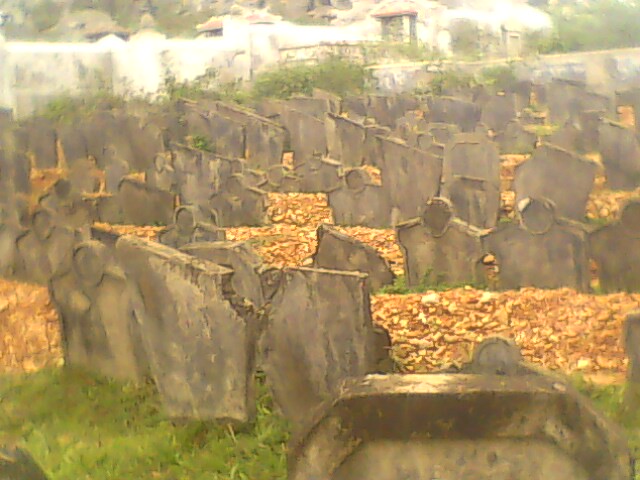The image depicts an antiquated graveyard with dozens of gravestones stretching from the front to the back. The scene is characterized by faded colors and blurriness, emphasizing its old and weathered state. The gravestones, mostly light gray with dark streaks and stains, share a uniform style and color. Many stones are uniquely sculpted to resemble humanoid shapes with rounded heads and visible shoulders, while others are more irregular and plain. The ground in the cemetery appears to be covered with light brown mounds or terraced rocks, adding to its aged look. In the background, beyond a wall, there are white buildings with red tile roofs and some greenery, including grass and trees, contrasting with the cemetery's somber tones.